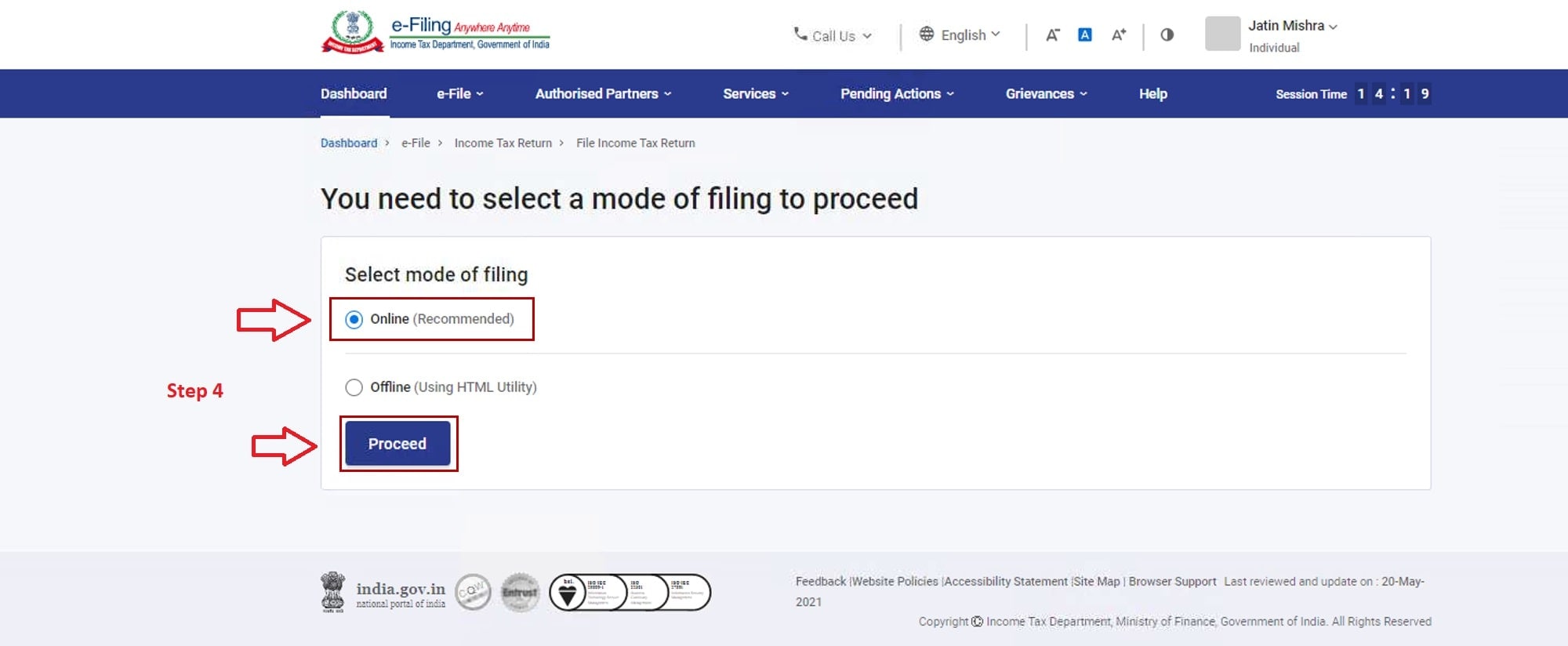Screenshot of an Indian Electronic Tax Filing Interface

The screenshot displays the user interface of India's electronic tax filing platform, as indicated by the logo "india.gov.in" situated at the bottom left corner. At the top, there's a circular blue logo with a red banner, though the white text on the banner is not legible. Adjacent to this icon, it reads "e-filing, anywhere, anytime" and is followed by "Income Tax Department, Government of India" in very small print.

A prominent blue banner stretches across the screen with white text listing various menu options: Dashboard (highlighted), e-file, Authorized Partners, Services, Pending Actions, Grievances, Help, and Session Time, which currently shows "14:19". Above this banner, set against a white background, are options to "Call Us," language selection ("Select English"), and text/font modification. The name "Jatin Mishra" appears prominently.

Below the darker blue banner, there's a pale blue background with a text box. Above this text box, a bold instruction states "You need to select a mode of filing to proceed." A red arrow points to a red-bordered text box labeled "Select mode of filing," offering the choices "Online" or "Offline," with "Online" currently selected. A blue "Proceed" button framed in a red text box is situated under the "Step 4" label.

The interface is designed to provide clear navigation and options for taxpayers to file their returns electronically, emphasizing user accessibility with options and clear instructions.